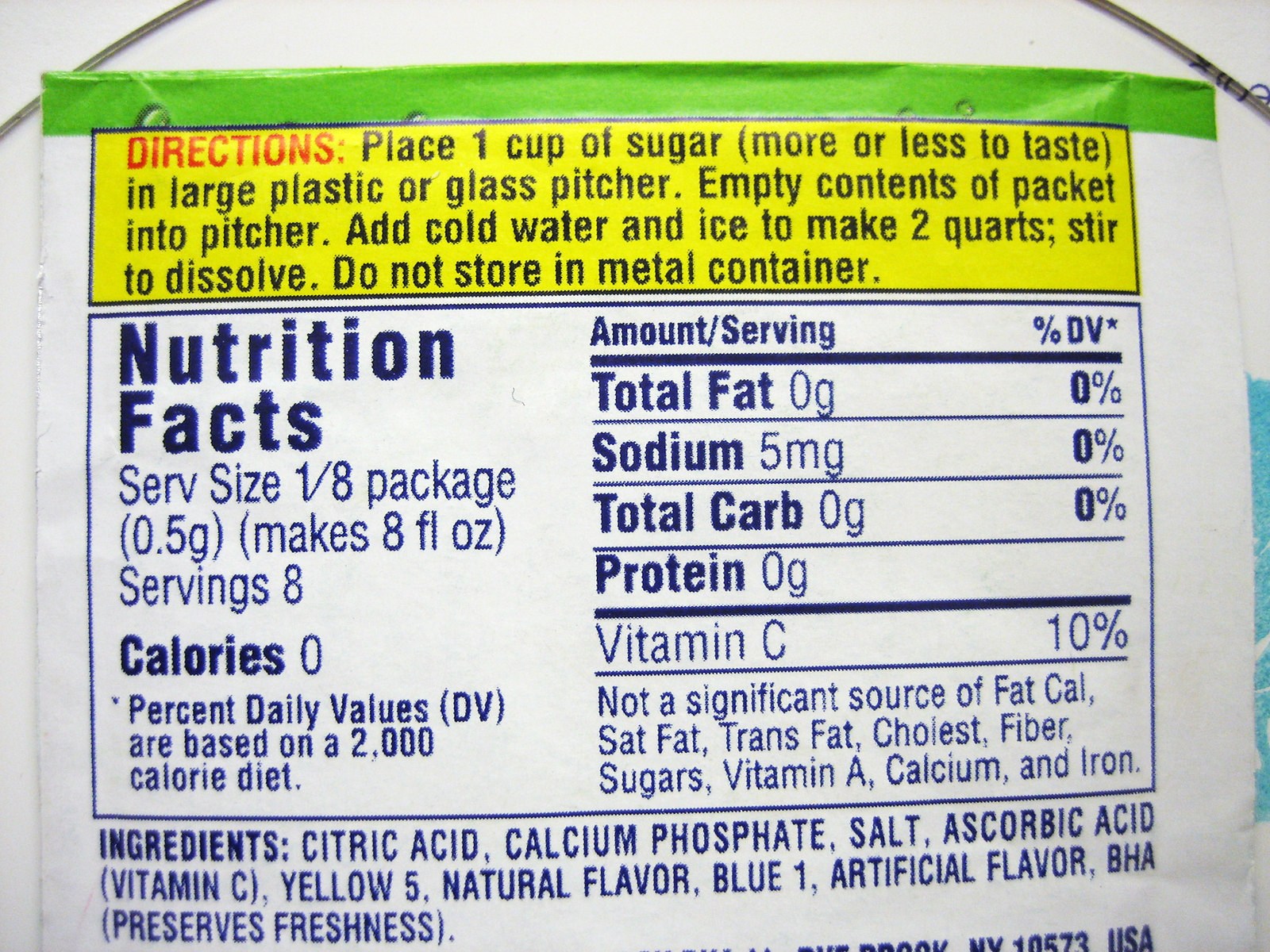This image features a detailed label on the back of a product package. At the top, there's a green strip followed by a yellow rectangle containing the preparation instructions. The instructions, written in black text dominated by a red "Directions" title, advise adding one cup of sugar (to taste) into a large plastic or glass pitcher. The packet's contents are then emptied into the pitcher before adding cold water and ice to make two quarts, stirring to dissolve. It's emphasized not to store the mixture in a metal container.

Below the directions, a white rectangle presents the "Nutrition Facts" in bold. The serving size is listed as 1/8 of a packet, making 8 fluid ounces per serving, with the package containing eight servings. Each serving has 0 calories. Detailed nutritional information includes 0 grams of total fat, 5 milligrams of sodium (0% DV), 0 grams of total carbohydrates, 0 grams of protein, and 10% DV of Vitamin C. A note clarifies that it’s not a significant source of calories, fat, trans fat, cholesterol, fiber, sugars, vitamin A, calcium, or iron.

At the bottom, the ingredients are listed in black text against a white background: citric acid, calcium phosphate, salt, ascorbic acid (vitamin C), Yellow 5, natural flavor, Blue 1, artificial flavor, and BHA for preserving freshness. The background of the label is predominantly white, with all the text featured in a black or bluish-black color.